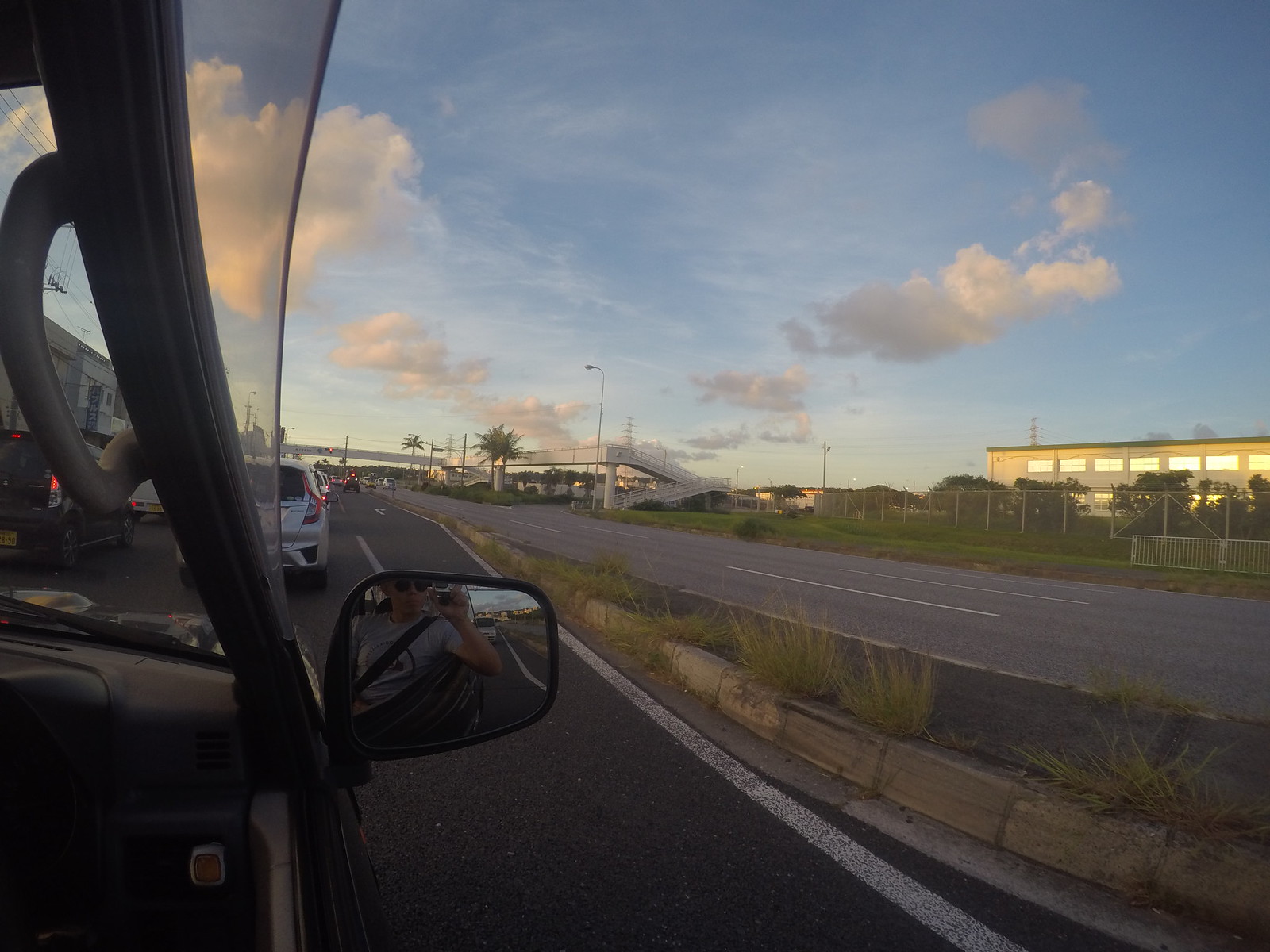Captured from the driver's seat, this photograph provides a dynamic view from inside a car while paused in traffic. The door frame and rearview mirror on the left side subtly frame the scene, adding context to the image. In the rearview mirror, a reflection reveals the photographer, holding a compact camera and aiming it out the window. The sky, bathed in the golden hues of an impending sunset, is adorned with clouds glowing warmly. The urban backdrop features buildings gleaming with the same golden light, emphasizing the time of day. Near the horizon, a pedestrian bridge and overpass span the highway, offering a sense of distance and scale. Ahead, several cars stand still on the road’s left lane, indicating a common traffic halt, adding a layer of everyday realism to the picturesque setting.